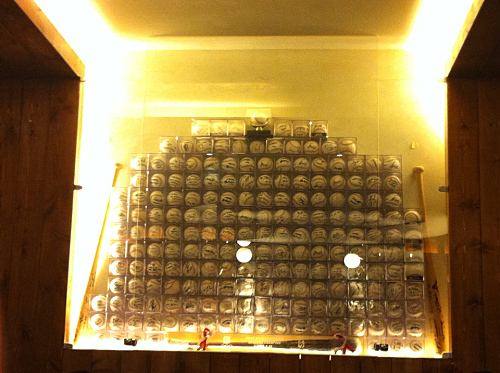This is a color photograph depicting a meticulously arranged display case containing numerous baseballs, each individually encased in small, transparent plastic cubes. The baseballs, likely signed though the signatures are not legible, are stacked in a grid-like pattern to form an impressive rectangular arrangement. The display is prominently lit by bright yellow lights situated at the edges, enhancing the visual appeal and contrast against the background. The case features glass on the front and appears to also include a baseball bat at its base. The photograph is framed by brown wooden doorways flanking the left and right sides of the image, which appear dark in comparison to the brightly lit display at the center. The setting is devoid of people, animals, plants, or any other objects, ensuring full focus on the carefully curated baseball collection. The background is a wood panel, adding a warm rustic touch to the scene.